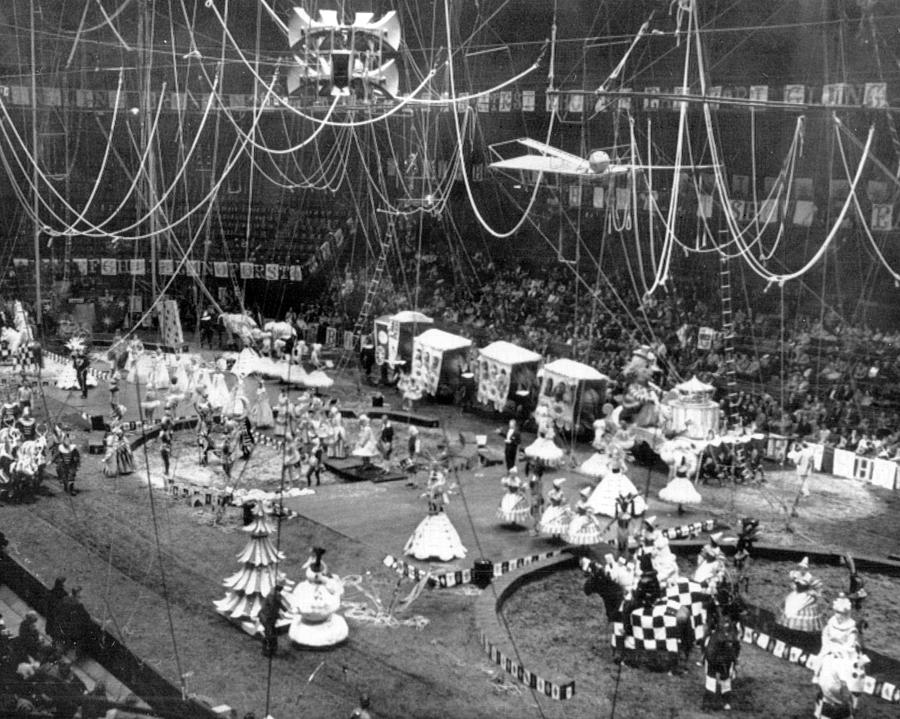This black-and-white photograph from the early 1900s or late 1800s depicts a bustling indoor circus scene, captured in its vintage grandeur. Suspended from the ceiling, numerous ropes and wires form scalloped patterns, possibly for acrobatic acts, adorned with loudspeakers overhead. The circus is staged in a large arena filled with spectators seated in the background, their attention captivated by the performances.

On the ground, two distinct entertainment rings are prominent, one on the left and another on the right, separated by an open area. Off to the left, a figure can be seen leading a group of animals, likely horses or donkeys, suggesting an ongoing parade or a preparation for the next act. In the back corner, angled carnival cars, reminiscent of gypsy wagons, add to the nostalgic ambiance.

Artists are positioned throughout, some wearing voluminous skirts, indicative of the period's fashion, possibly preparing for or engaging in a performance. In the center ring, one performer, donned in a black suit with a white front, likely the ringmaster, stands out prominently. Additional details include scattered ladders reaching up towards the ceiling and a miniature train setup contributing to the circus's elaborate staging. Banners with indistinguishable letters hang on the left side near the audience, adding to the festive yet antique atmosphere of this crowded, lively scene.